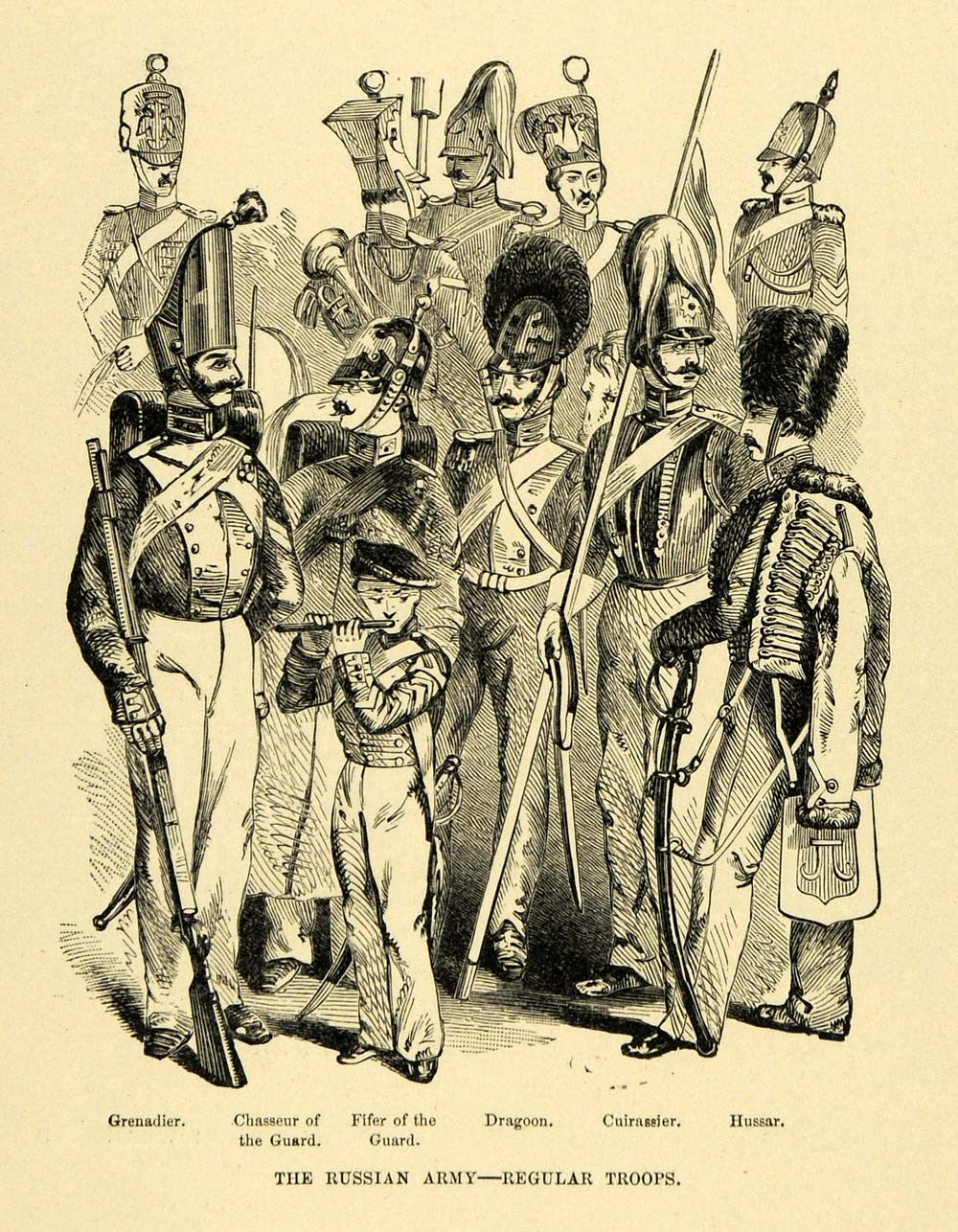An aged, hand-drawn black and white ink illustration, likely from the 1700s or 1800s, depicts a group of Russian soldiers. The drawing, rendered on yellowing paper with a very light brown background, features thin, meticulous pen strokes. The soldiers are dressed in elaborate military uniforms, with some donning tall, feathery hats adorned with floral or star-like emblems, while others wear round black hats. The men in the foreground carry various weapons, including muskets, swords, and flags, although the flag details are indistinguishable. Among the soldiers, a young boy stands out, wearing a military uniform with a beret and a holstered sword, playing a flute. Beneath the illustration, text identifies the soldiers as regular troops in the Russian Army, listing their roles: Dragoon, Pfeifer of the Guard, Chasseur of the Guard, Curassier, and Hussar.